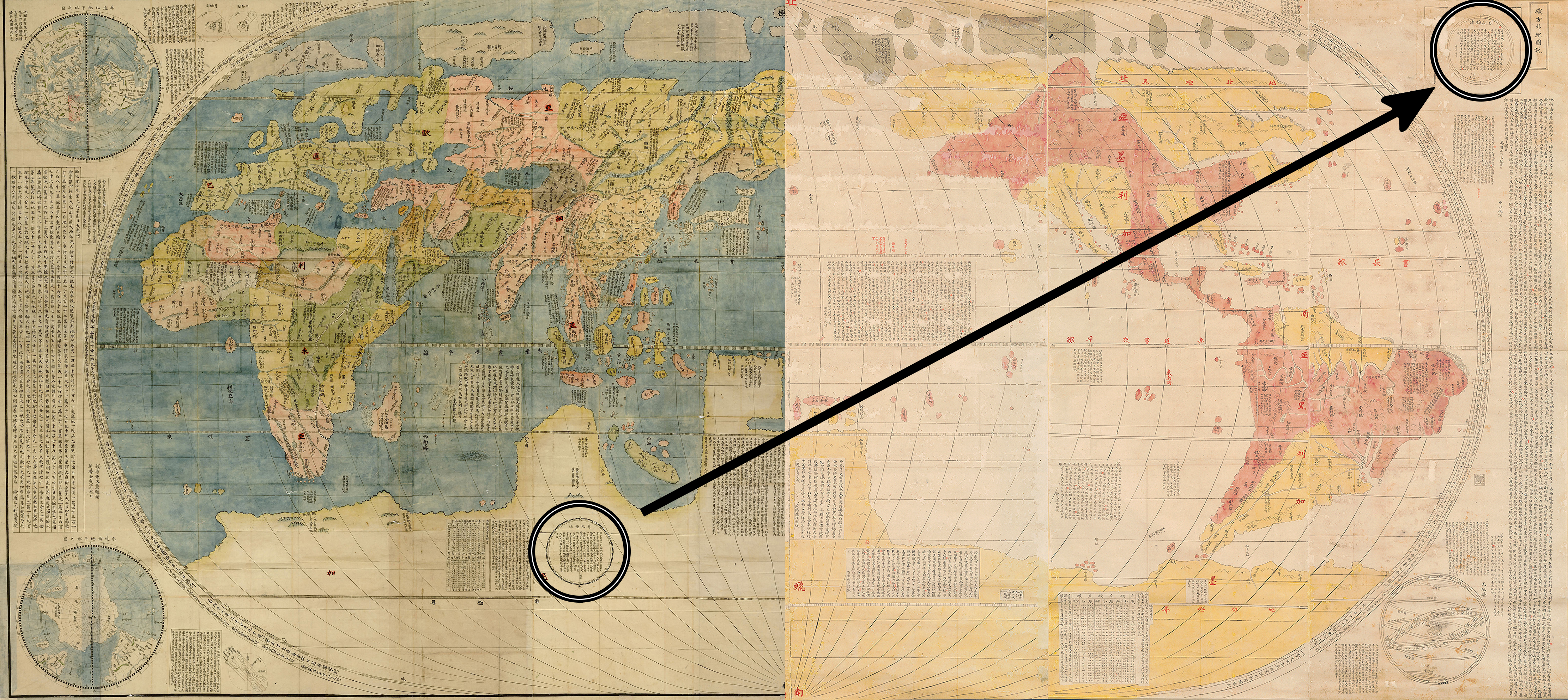This photo showcases a large, detailed world map split into hemispheres, appearing almost as if two different maps have been juxtaposed. The left side features a brightly colored, traditional map with blue oceans and landmasses in green, red, and yellow, ranging from Africa to Asia. This side also includes intricate and small yet legible text. The right side contrasts with a more muted color scheme, displaying North and South America in reds and yellows, with notable open and solid black circles connected by a long black arrow pointing from the left hemisphere to the right. Numerous small scripts and additional circles are present across both halves of the map, adding to the rich detail and complexity of the visual.